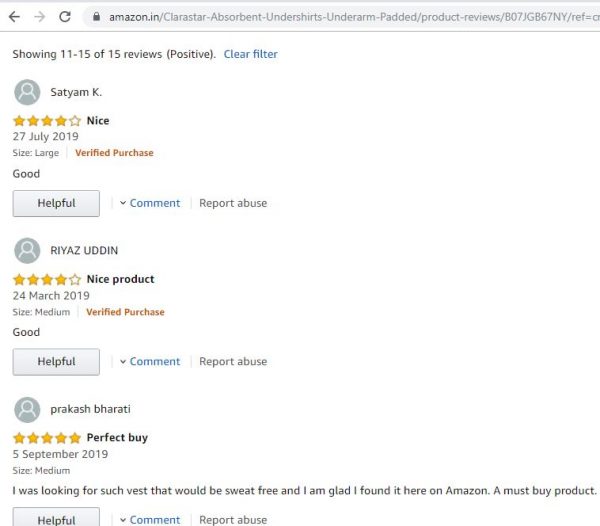This is a detailed screenshot of Amazon reviews from Amazon India for the product page of "CLARSTAR Absorbent Undershirts Underarm Padded." The browser address bar at the top reads: "amazon.in/CLARSTAR-absorbent-undershirts-underarm-padded/product-reviews/B07JGB67INY/ref=..." followed by an unreadable portion. 

The page shows reviews 11 to 15 out of 15, filtered to display positive feedback first. 

1. Review by "Satyam" – Rated 4 Stars.
    - Posted on: 27th July 2019.
    - Review: One word, "Good."
    - Purchase details: Size Large, Verified Purchase.

2. Review by "Riyazuddin" – Rated 4 Stars.
    - Posted on: 24th March 2019.
    - Title: "Nice Product."
    - Review: Brief comment, "Good."
    - Purchase details: Size Medium, Verified Purchase.

3. Review by "Prakash Bharati" – Rated 5 Stars.
    - Posted on: 5th September 2019.
    - Title: "Perfect Buy."
    - Review: "I was looking for such a vest that would be sweat-free and I am glad I found it here on Amazon. A must-buy product."
    - Purchase details: Size Medium, Verified Purchase.

Each review includes options to mark it as helpful, add comments, or report abuse at the bottom.